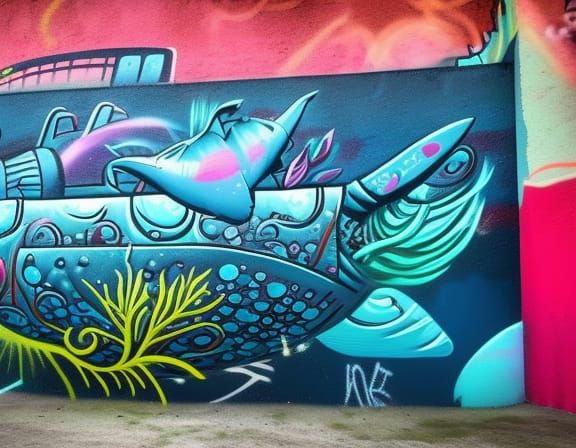The image depicts a vividly detailed mural that covers the entirety of a wall. The dominant feature is a large midnight blue rectangle that occupies most of the mural, set against a backdrop of red spray paint interspersed with various colors such as green and yellow. The mural's upper section features swirls of red and yellow lines. 

The focal point within the blue rectangle includes intricate designs resembling coral, executed in purples and greens to give the illusion of different textures. Specifically, in the lower left corner, a bright green vine-like structure is prominently visible.

To the left side of the mural, there is a striking yellow, elongated plant-like object that ascends vertically. Adjacent to it, portions of the design appear to resemble abstract shapes that could be interpreted as mechanical or underwater elements, such as a flashlight, a car, or submersible creatures, rendered in teal greens and pinks. Further down, towards the bottom of the mural, there are teal circular and linear designs that appear bowl-like.

The mural's right section includes a patchwork of colors—red, white, and pink—alongside rock-like structures in teal hues. Below these structures, there is some sort of ambiguous writing that resembles Asian characters but isn't clear. The entire artwork is set against a sidewalk with a pattern of gray and black splotches, adding to the dynamic and eclectic nature of the scene.